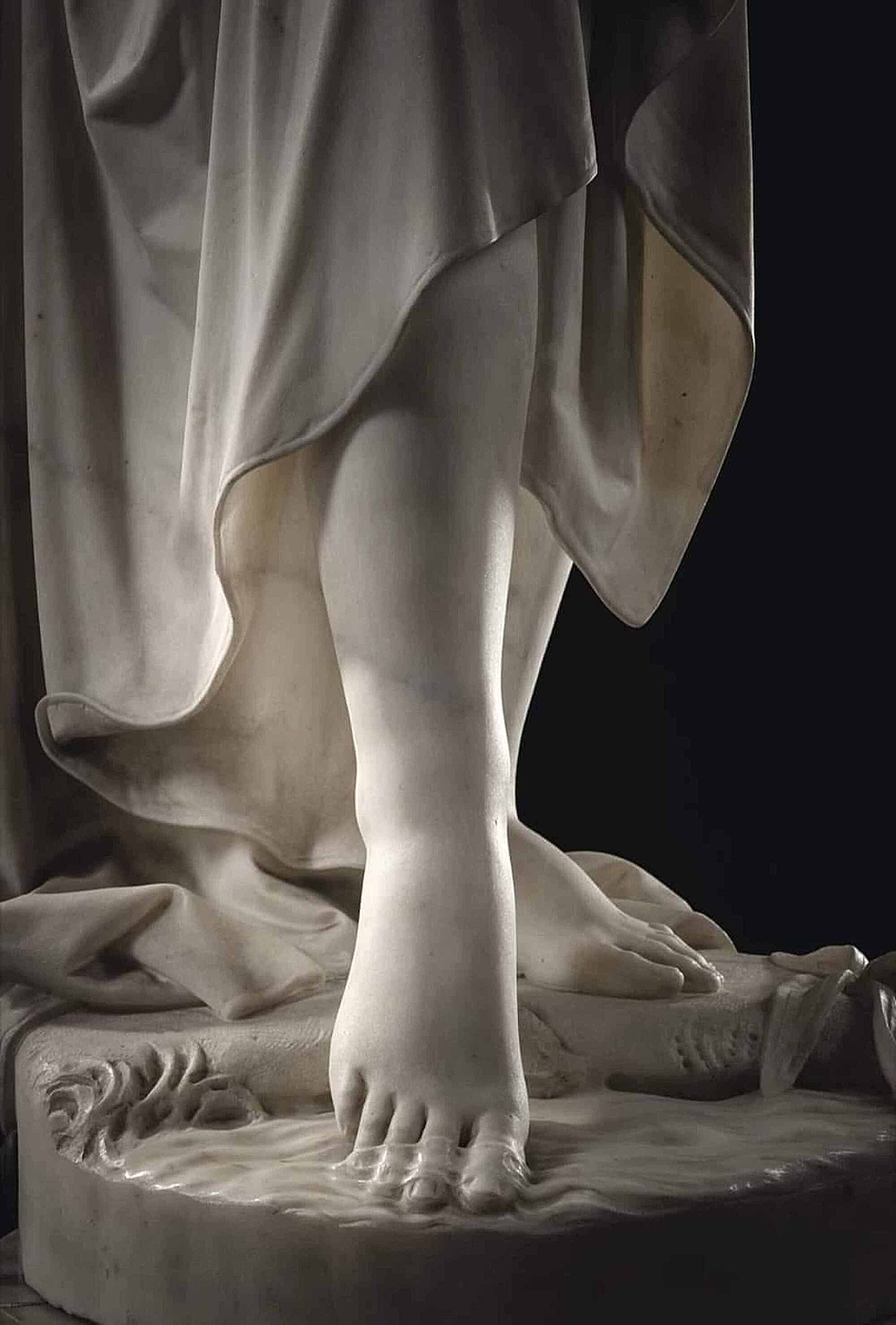The image depicts a close-up of the lower legs and feet of a white marble statue, set against a completely black background. The statue appears to be female, characterized by its smooth, medium-sized legs and flowing garments. The figure's left foot is arched and submerged in a realistic depiction of shallow water, with water flowing over and around the toes, creating a glistening effect. This foot is placed on a slightly lower, rocky surface. The right foot, placed on a higher platform, is flat and partially covered by a transparent section of the robe. The dress or robe drapes elegantly down to just below the knee, with its hemline revealing a mix of intricate marble folds that simulate fabric. The careful carving and fine details enhance the lifelike appearance, making the stone attire seem like fluid cloth. A small portion of the robe pools behind the feet on the base, adding to the realism. No signatures or text are visible on the statue.